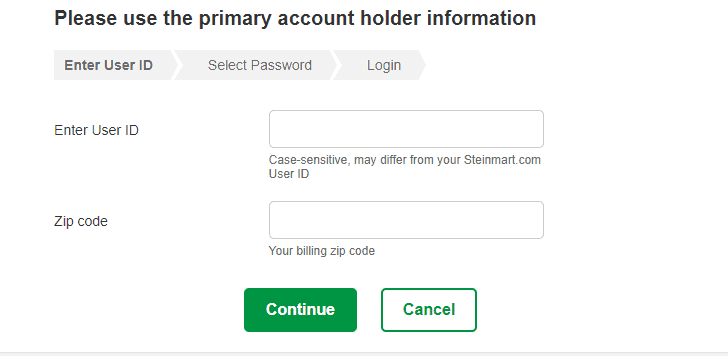The webpage interface presented for logging into the primary account contains the following elements arranged in an organized structure:

1. **Primary Account Login Section**:
   - **Instructional Text**: A text prompt on the left that reads "Enter User ID."
   - **Input Field**: To the right of this text is a bar for entering the user ID.
   - **Note**: Below the input field, in gray, it states "Case sensitive, may differ from your steinmark.com user ID."

2. **Billing Information Section**:
   - **Instructional Text**: On the far left, it says "ZIP Code."
   - **Input Field**: To the right of this text is a bar for entering the billing zip code.
   - **Note**: Below the input field, it instructs "Your billing zip code."

3. **Action Buttons**:
   - **Continue Button**: Centrally placed, a green select button labeled "Continue."
   - **Cancel Button**: Next to it, a hollowed-out button with "Cancel" in green text.

4. **Additional Information**:
   - **Instructional Text**: There’s a reminder in gold and black that reads, "Please use the primary account holder information," suggesting that the primary account holder's information should be utilized for login.

5. **Page Layout**:
   - There is a clear progression with minimal white space that maintains a clean, organized appearance, with green and white elements driving attention to the action buttons.

In summary, the design aims to create an intuitive and straightforward user experience, directing attention to the critical sections required for logging into a primary account, and clearly marking sections with relevant, concise instructions.